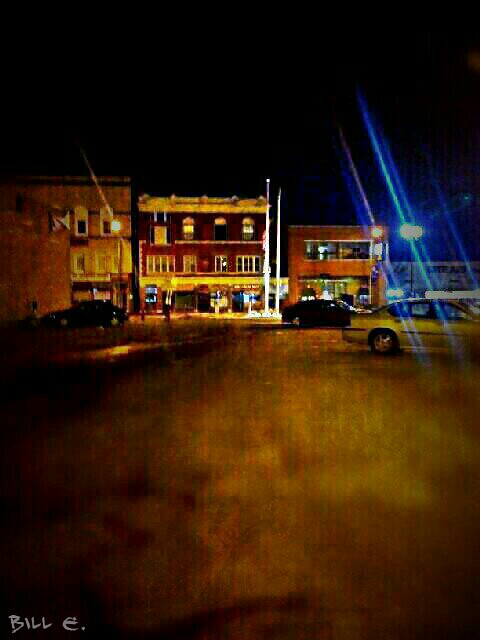This nighttime image captures a blurry street scene, dominated by a pitch-black sky and an out-of-focus parking lot with several cars. In the foreground, there are a couple of parked cars: one is silver and another is black. Another car, either gray or yellow, appears to be driving by. To the left, there is a red three-story brick building with its lights on, accompanied by lighter brown brick buildings. The right-hand side showcases a mix of brown and white buildings decorated with white poles bearing American flags. Streetlights are visible on the right, emitting a blue glare against the dark sky. A small billboard is located to the far right, and at the bottom left corner of the image, the name "Bill E." is subtly inscribed.